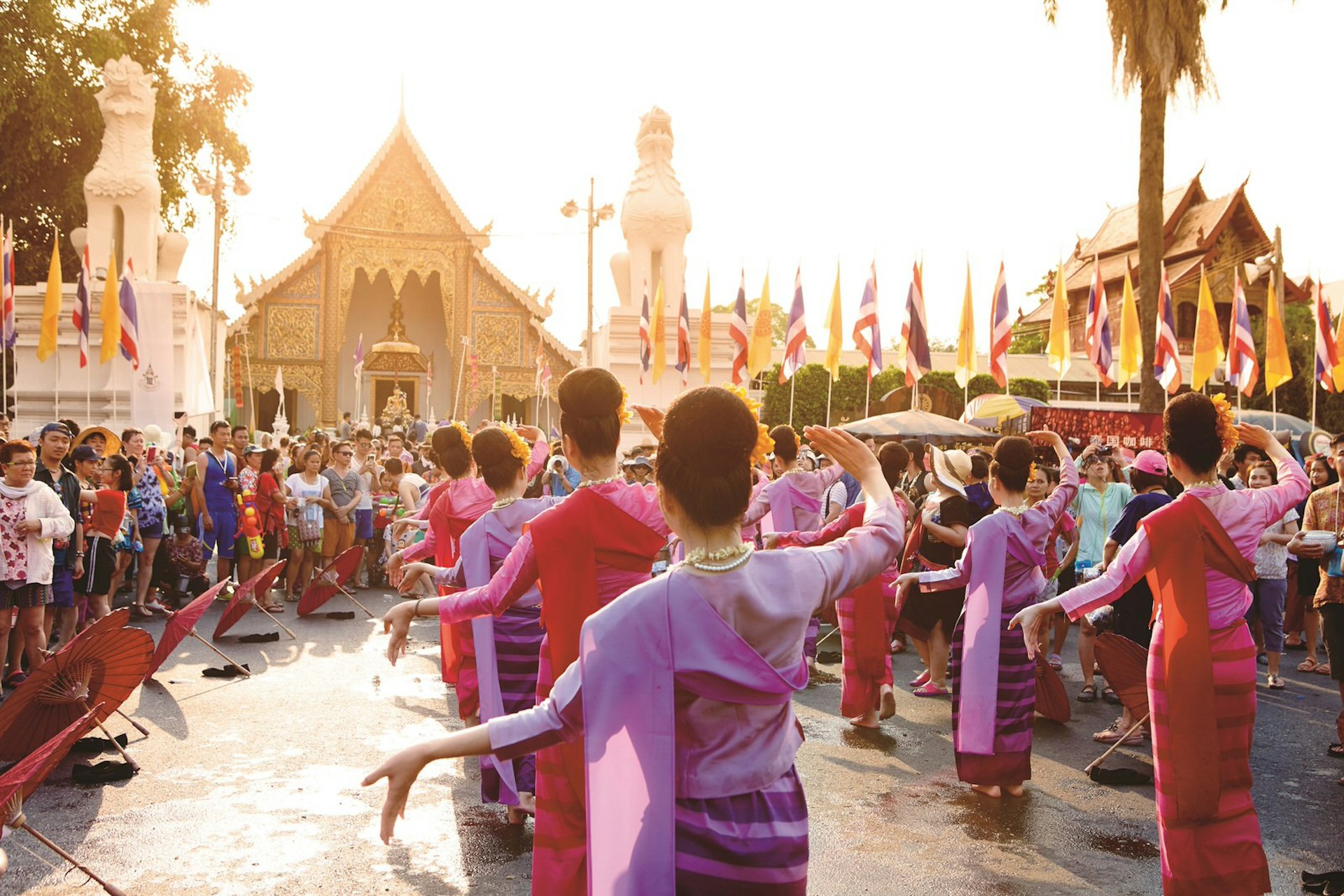The photograph captures an outdoor ceremony in the center of a foreign town, likely located in Asia, possibly China or Southeast Asia, during sunset. In the heart of a bustling town square, eight women, dressed in alternating red and purple gowns with sashes, perform a synchronized dance. Their movements are precise, with their left hands extended outward and right hands raised near their heads. Each dancer has her hair intricately styled in a high band. Surrounding the performers is a large, captivated crowd, possibly over a hundred onlookers, dressed in summer attire, indicative of warm weather. Scattered on the ground are colorful umbrellas, suggesting they were used in a previous segment of the routine. The background features tall structures and statues, resembling traditional Chinese or Japanese architecture, including what might be a dragon sculpture, enhancing the cultural ambiance of the scene.